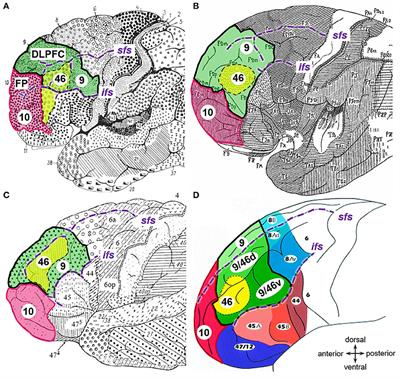This is a detailed description of a diagram divided into four sections labeled A, B, C, and D, which appears to depict developmental stages, potentially of a brain or an embryo. Each section displays curled, embryo-like figures with specific regions colored in pink, green, yellow, and various other hues, while the rest of the figures remain in black and white. 

Section A features light shading and spotting. Section B is rendered much darker with extensive gray areas. Section C offers a closer view, highlighting a green spotted area along with distinct yellow and red parts. Colored regions in these sections are numbered and labeled, featuring terms such as SFS and LFS.

The figure in Section D, located in the bottom-right corner, displays an array of colors including green, yellow, and blue, indicating more detailed or advanced features. Additionally, there is a compass-shaped icon in the corner, annotated with 'dorsal,' 'anterior,' 'ventral,' and 'posterior,' each word aligned with a corresponding direction.